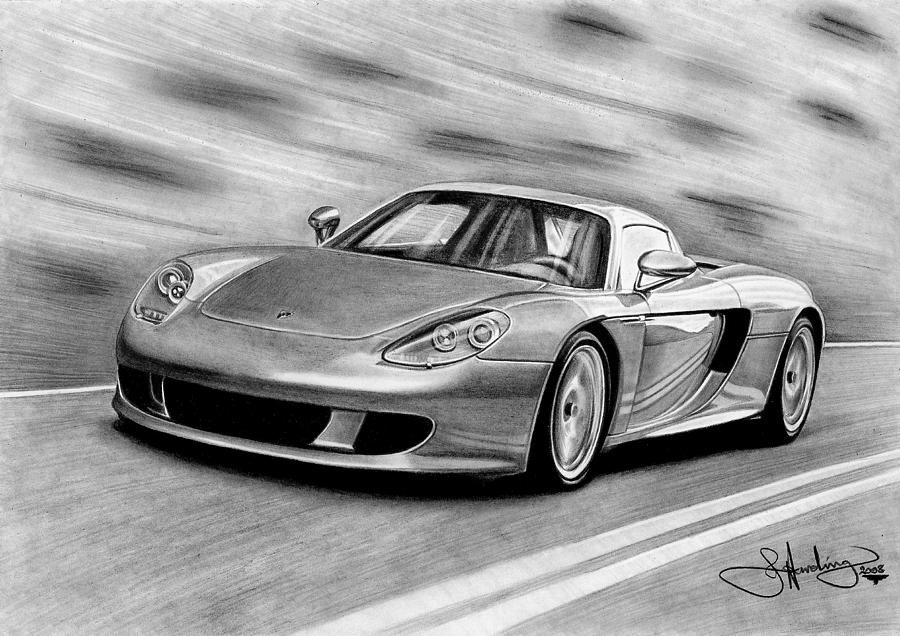This image is a detailed, black and white illustration created with charcoal, graphite, or pencil, capturing a high-speed sports car on a paved highway. The grayscale drawing depicts a sleek, two-seater car that resembles a Ferrari or Porsche, positioned on the right side of a double-striped road. The car is oriented slightly to the left and appears to be in motion, emphasized by a background blur effect that suggests high speed. Notably, the car lacks a visible driver, revealing only empty bucket seats through its windshield.

The drawing is presented in landscape orientation and features reflections on the car's side, highlighting its metallic sheen, despite the monochrome palette. The lower right corner bears the artist's signature, which seems to start with an 'S' and possibly ends with 'Harding,' followed by the year 2008. The entire composition effectively conveys the thrilling dynamism of the car speeding down the highway.